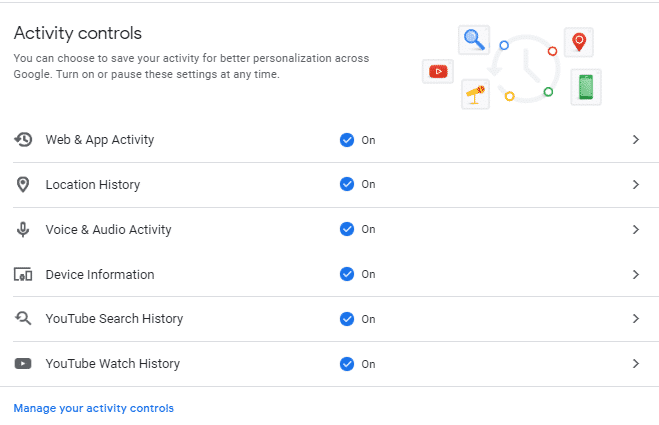This image is a detailed screenshot of the Google "Activity Controls" page, primarily relevant to YouTube. The screenshot showcases a standalone window with a minimalist white background and a faint gray horizontal line near the top.

At the top left, the text "Activity Controls" is prominently displayed in bold black font. This section explains that users can choose to save their activity for improved personalization across Google services and can toggle these settings on or off at any time.

To the right is a stylized clock icon in light gray, featuring colored dots at each quarter: a blue dot at 10 o'clock, an orange dot at 2 o'clock, a green dot at 5 o'clock, and another orange dot at 7 o'clock. Surrounding this clock are five gray-outlined square icons: an orange pen, a green cell phone, a yellow telescope, a red play button, and a blue spyglass.

Below this header, a list of activity settings is presented, each separated by a pale gray line. The settings are listed as follows:

1. **Web and App Activity** - This setting is turned on, indicated by a blue icon with a white check mark to the left, and a forward gray arrow on the far right.
2. **Location History** - Similarly formatted with its respective icon and a forward gray arrow.
3. **Voice and Audio Activity** - Following the same format.
4. **Device Information** - Similarly structured.
5. **YouTube Search History** - Following the same layout.
6. **YouTube Watch History** - Conforming to the same design.

Each setting line features corresponding icons to the left of their titles: a clock, a pen, a microphone, a computer monitor, a search glass, and a YouTube play button.

At the very bottom, below the final gray line, a blue link reads "Manage Your Activity Controls," guiding users to further manage their settings.